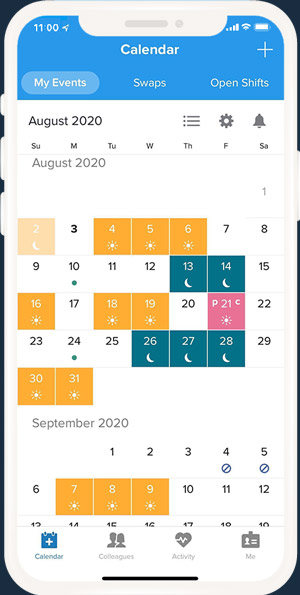Here is a detailed and cleaned-up caption for the image:

"A white mobile device is displayed against a black background. On the left side of the device, the volume up and down buttons, as well as the power button, are visible. The screen of the device shows a calendar application. The top portion of the screen has a blue background, with a plus symbol in the top right corner and the word 'Calendar' prominently centered. Below this, there are tabs labeled 'My Events,' 'Swaps,' and 'Open Shifts.' The main calendar interface has a white background and is labeled 'August 2020.' This section also features buttons for list view, settings, and a notification bell icon. The calendar grid displays days from Sunday to Saturday. Several dates are marked with colored tiles – orange for day shifts, greenish-blue for night shifts, and one pink tile, which might indicate a special event or an outlier. This detailed setup is neatly organized for easy navigation and viewing of scheduled events."